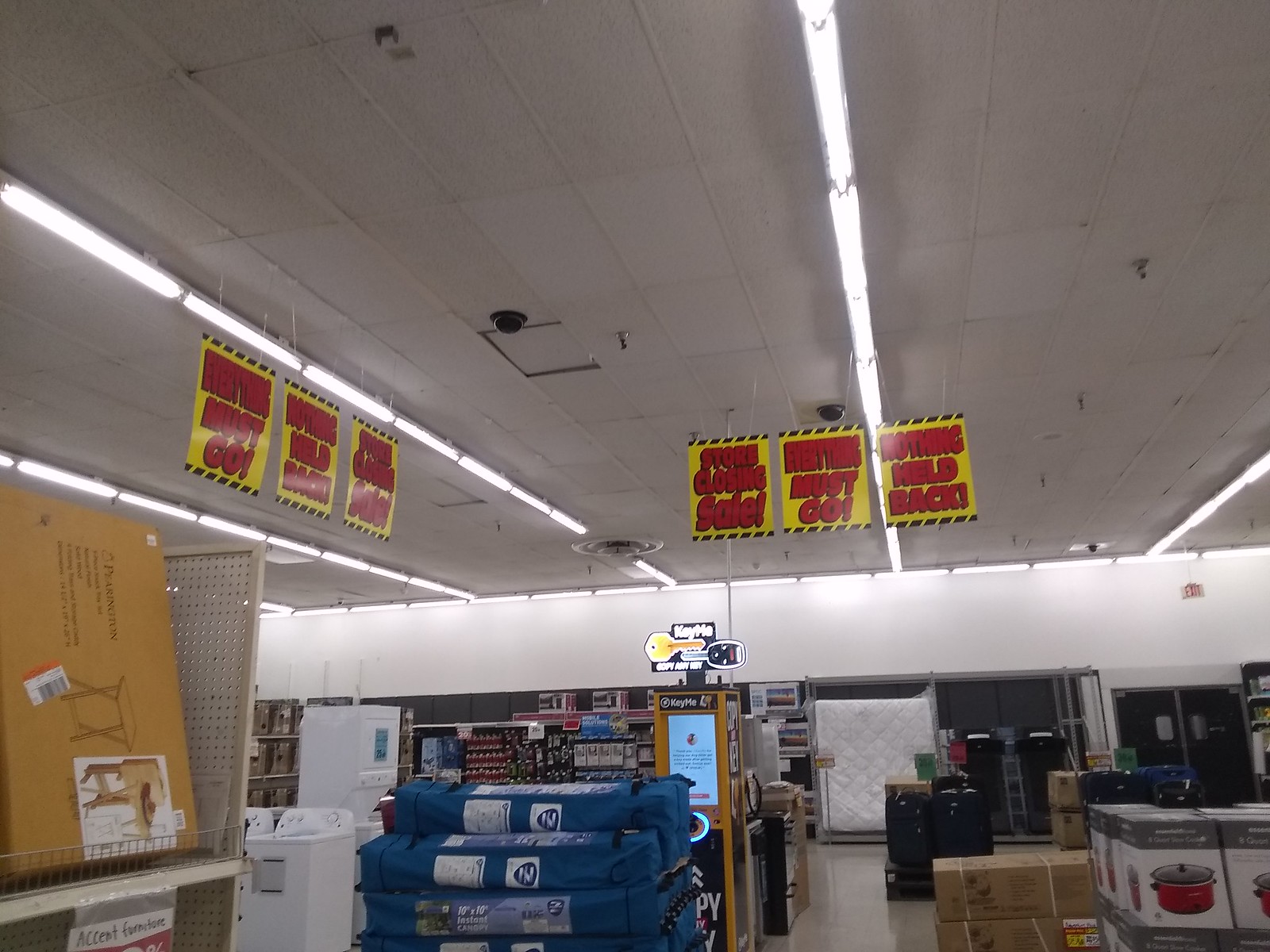This is a detailed photograph taken inside a retail store, likely a discount or closing sale establishment. The store features an acoustic tile ceiling with multiple rows of fluorescent lighting strips. Prominently, there are yellow signs with red text hanging in pairs of three from the ceiling, declaring "Store Closing Sale," "Everything Must Go," and "Nothing Held Back."

On the left side of the image, there's a shelving unit hosting a boxed TV tray. Nearby, a pallet is stacked with collapsible outdoor canopies, and next to it, there’s a key-cutting kiosk labeled "Keys Made" or "Key Me." Further along, towards the back, you can spot washing machines and other large laundry appliances.

At the center of the image, a pile of blue duffel bags occupies the floor space. In the right bottom corner, boxes of slow cookers are visible, with what appears to be luggage or additional duffel bags situated behind them. The background displays various items extending towards a stark white wall, punctuated by a solitary mattress positioned against it. The store’s utilitarian setup is accentuated by the utilitarian fluorescent lighting and commercial ceiling vents.